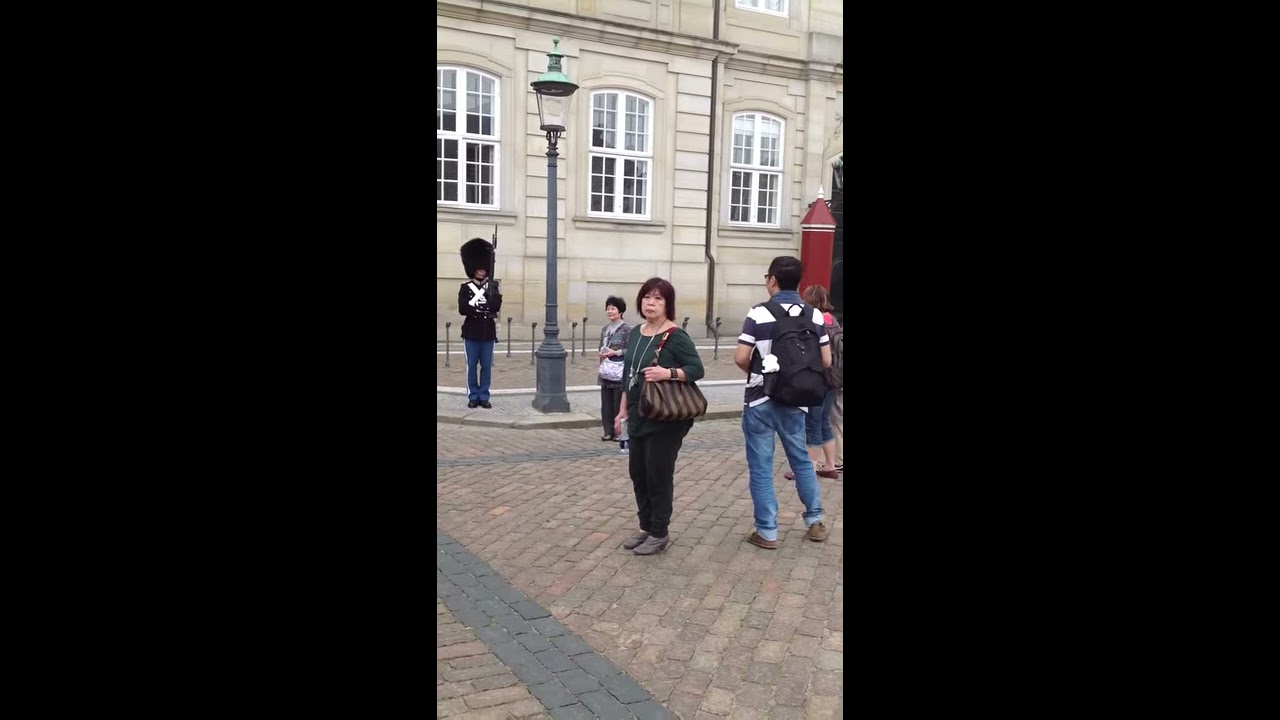This outdoor photograph, likely taken by a tourist, captures a scene set against a cream-colored brick building with white or light gray paned windows. The area outside the building is paved with rectangular bricks, primarily brown with patterns formed by some black bricks. In the front and center of the photograph stands an older Asian woman with medium-length black hair cropped at her shoulders. She is wearing a frumpy dark round-necked blouse, black pants, and gray boots. With a neutral expression, she holds a vertically striped brown handbag over her left shoulder, her left arm bent at the elbow resting on the bag.

Directly behind her, a tall wrought iron lamppost stands unlit in the daylight. To her left, near the edge of the building, a prominent sentry is stationed. The guard is dressed in a tall fur hat, a black military coat, blue pants, and is holding a rifle. In the background, another woman and a young man are visible. The young man, facing the building, wears a black and white striped t-shirt, blue jeans, dark gray sneakers, and a black backpack. A tall red door, possibly the building's entrance, is noticeable on the right side of the image near the corner of the building.

Framing the image on the left and right are two vertical black strips, giving the photograph a tall and skinny appearance, as though it might have been taken on an iPhone. The overall scene depicts a bustling yet historical atmosphere, with individuals observing the setting, possibly in the UK, as suggested by the presence of the sentry in traditional ceremonial attire.